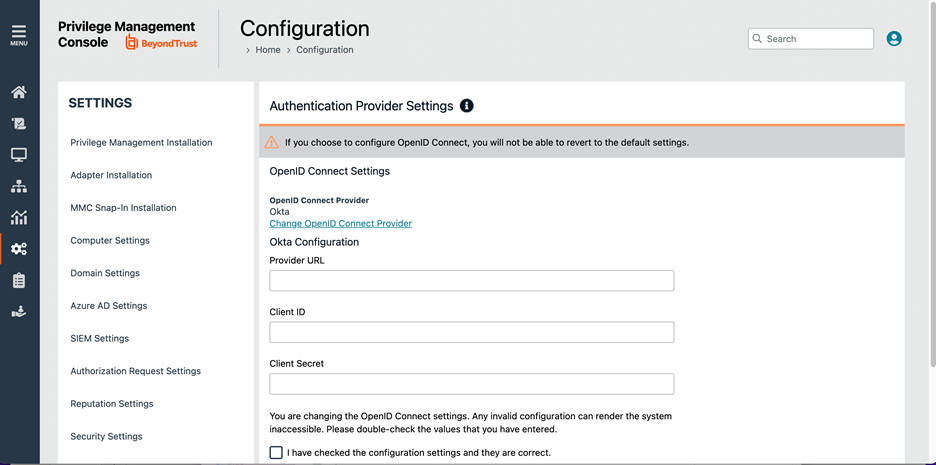The image depicts a detailed interface of a privilege management console set against a white background. At the top, there is a home configuration option alongside a search bar, represented by a magnifying glass icon, and a profile icon showcasing a gray human figure on a blue background.

On the left side, a blue sidebar contains a hamburger menu icon that expands to reveal a comprehensive menu. This menu includes settings for various configurations such as:
- Privilege Management Installation
- Adapter Installation
- MMC Snap-in Installation
- Computer Settings
- Domain Settings
- Azure AD Settings (where "AD" is in capital letters)
- SIEM Settings (with "SIEM" in all caps)
- Authorization Request Settings
- Reputation Settings
- Security Settings
- Authentication Provider Settings

Additionally, the interface displays a notable black circle featuring a white eye icon, indicative of a surveillance or monitoring function. There is also a prominently placed caution icon warning users that opting to configure OpenID Connect will disable reverting to default settings.

For OpenID Connect settings, there is reference to setting up an OpenID Connect provider, with examples such as "Okta" (with "Okta" appearing as a blue hyperlink). Options under this section include changing the OpenID Connect provider and Okta configuration details.

The overall interface is thoughtfully organized, providing an array of settings for a robust and secure privilege management system.